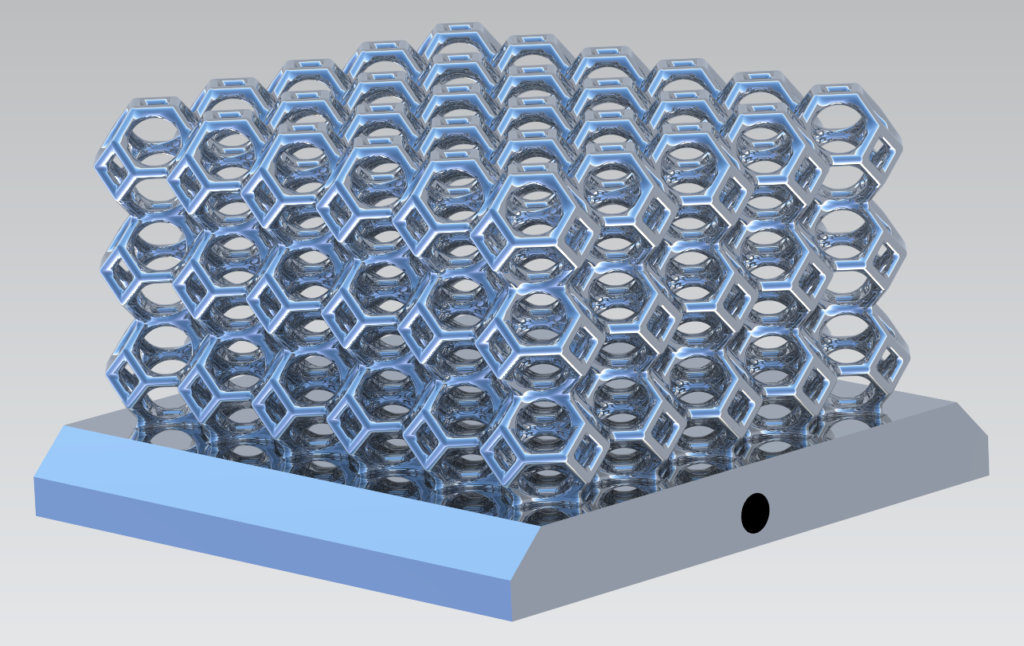The image appears to be a highly detailed digital rendering, possibly created using vector or CAD software, featuring a geometrically intricate structure. The central focus is a cluster of three-dimensional silver hexagons, arranged in a beehive-like formation, with approximately ten rows, each containing three or four hexagons. These hexagons are nested together to form a complex rectangular shape that rises from a square base. This base transitions from silver to shades of light and dark blue and sits on a light gray gradient background. One corner of the square base points towards the center of the image, while the other edges extend outwards. A prominent black circle is situated on the right side of the base, adding to the futuristic aesthetic of the scene. The entire composition, including the base and hexagonal structure, has a realistic yet computer-generated appearance, suggesting it is an artistic or conceptual design rather than a physical object.